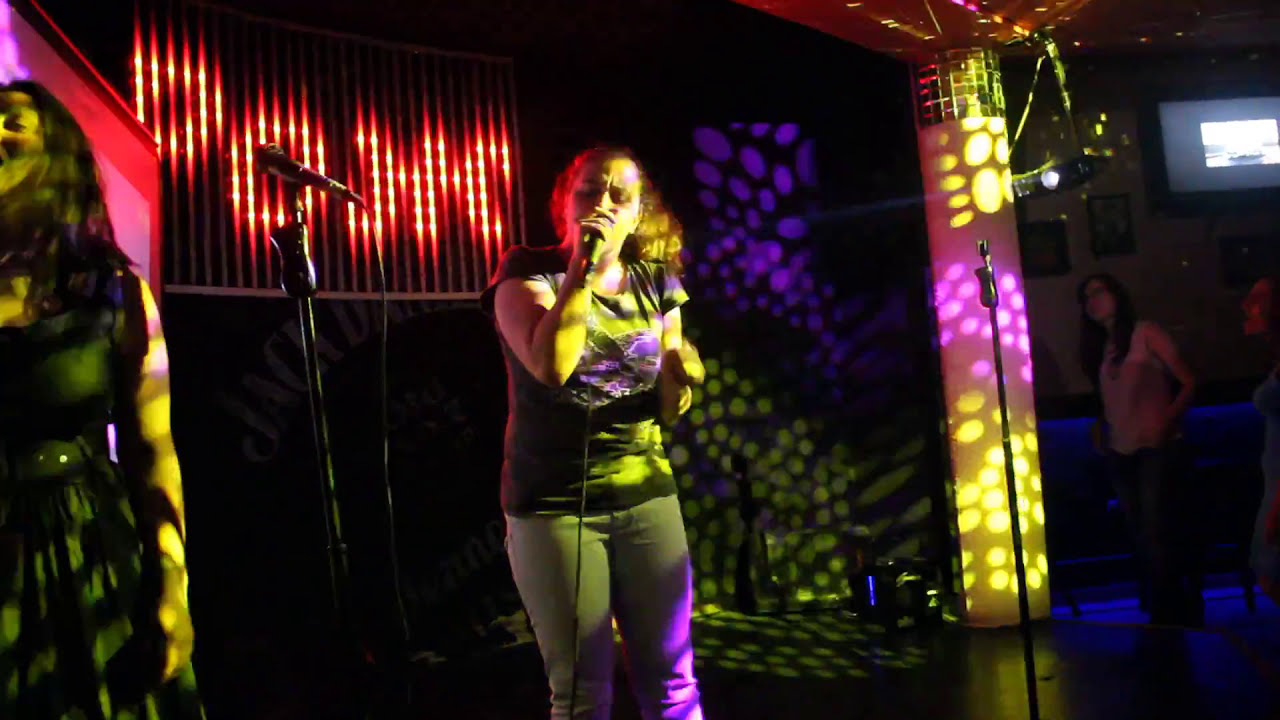This image captures a vibrant, indoor scene at a bar or karaoke club, likely in the evening. A rectangular stage is centered in the composition, where multiple women are performing. The central figure, a white woman, is deeply engrossed in her song, holding a microphone to her mouth with her eyes closed. She is wearing a dark t-shirt with screen printing and gray pants, and her hair is pulled back. To her left, partially visible, is another woman with long dark hair, dressed in a black sleeveless dress, also singing with closed eyes and head tilted back. The stage is dramatically lit with an array of colors including purple, green, yellow, orange, red, and pink, which creates a lively atmosphere. Behind the performers, there are strings of lights and possibly neon signs contributing to the dynamic backdrop. Off to the right of the stage, patrons of the bar can be seen, along with a woman standing who might be monitoring the performance or simply watching. The background also features a television screen, adding to the sense that this is a public entertainment venue. Various lighting elements hang from the ceiling, projecting patterned spots of color onto the stage, enhancing the overall mood.